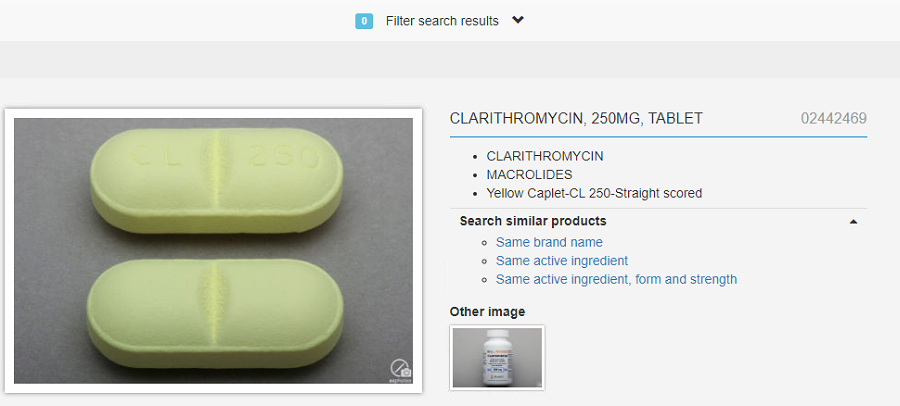In the image, the central focus is a user interface element for filtering search results. At the top middle, a bold heading reads "Filter Search Results." Directly to the left of this heading is a small, blue square containing the number "0." To the right of the heading, there's a black downward arrow icon.

Below this heading, to the bottom left, there's a large boxed area featuring a close-up photograph of two pills. The pills are similar in appearance, seemingly flipped upside down to reveal both sides. They are primarily yellowish with a distinct bright yellow area in the center. The top pill is embossed with the numbers and letters "CL-250," and both pills rest against a grayish background.

On the upper right side of the image, text reads: "Larry Thorman 250mg tablet." Adjacent to this text, there is a space followed by the code "0244-2469," both of which are underlined by a blue line. Below this, three bolded points are listed: the first point reads "Clarithromacin," the second reads "Marsalide," and the third reads "Yellow Caplet."